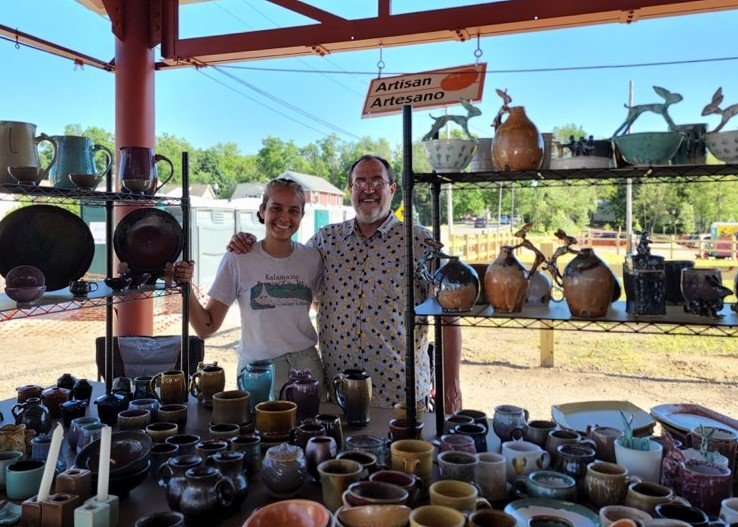In the photograph, a smiling man and woman are standing in front of a bustling pottery stall under a bright blue sky. The table in front of them is filled with an array of pottery, including coffee mugs, pitchers, plates, and tapered pots, all in varying shapes, sizes, and colors. The man, who has balding hair, a white beard, glasses, and a blue button-up shirt adorned with black dots, has his right arm comfortably resting on the woman’s shoulder. The woman, with her hair up in a bun and wearing a white t-shirt with a blue design, has her right hand holding a metal rack filled with additional pottery items. Above them, a sign reads "artisan, artisano" in black text on a white background, accented with an orange border and a circular orange in the top right corner. Behind them, a line of trees creates a serene backdrop, blended with glimpses of buildings and cars on either side, emphasizing the outdoor market setting.